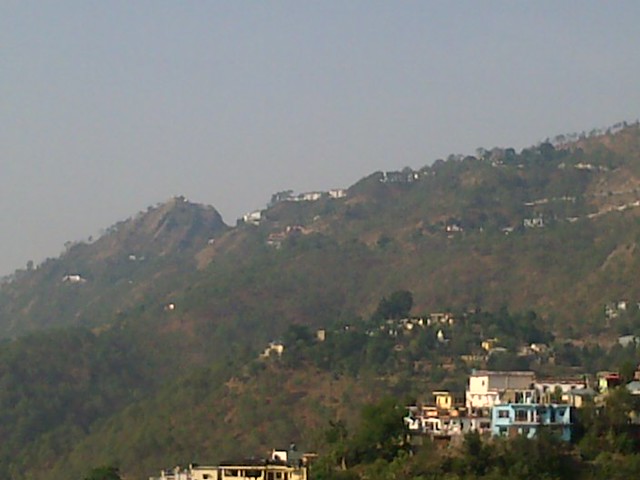The image captures a steep, rocky hillside that resembles a low-lying mountain, possibly located in a valley or coastal area. The scene is taken from a low-angle, roughly half a mile away from the base of the hill, accentuating its incline and making the foreground blend seamlessly into the background. The hillside is lush with a mix of dense trees, vegetation, and rocky outcroppings, which add texture and natural beauty to the landscape.

Prominently featured throughout various terraces on this hillside are clusters of homes, suggesting a possibly affluent neighborhood. At the very bottom of the scene, there is a striking yellow house situated on a terrace. Ascending about 200 yards above this yellow house are groups of terraced homes, including blue and white houses, which weave their way up the hillside. A few hundred feet beyond this group lies another plateau dotted with more terraced houses. Higher up, the hill levels off into a ridge, where distant houses can be seen, though they appear blurred by the expanse and the intermingling foliage.

Above this ridge, some homes perch atop the crest, silhouetted against a clear blue sky with no clouds in sight. The sky occupies the upper two-thirds of the image's left portion, while a purplish-blue hue suggests either early morning or late afternoon light. Despite the clear sky, the photograph has a slightly overcast feel due to its blurry and grainy texture. The overall scene is dynamic with an alternating pattern of natural landscape and human habitation, giving an intricate, tiered look to the hillside.